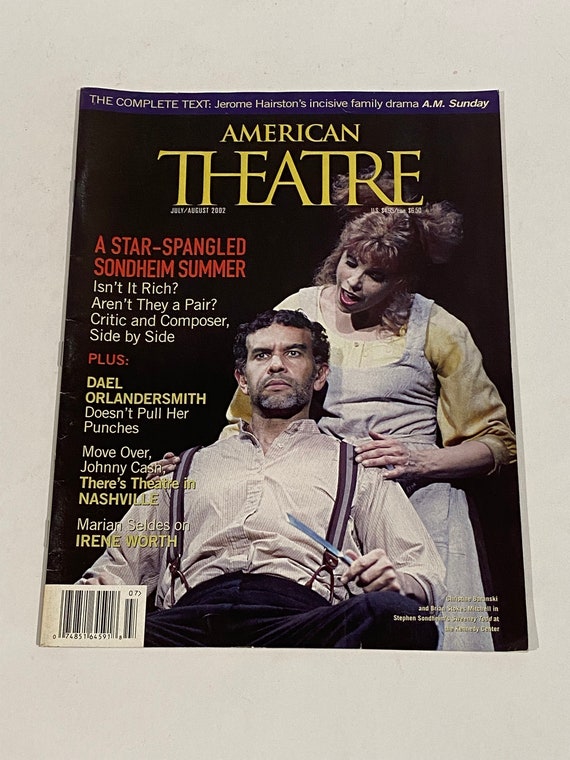The cover of the magazine "American Theater," dated July/August 2002, features a striking image of two individuals. The man, with short hair, a graying beard, and a slightly disgruntled or concentrated expression, is seated and holds a metallic knife in his hand, which adds an ominous tone to his demeanor. He is dressed in a light-colored button-up shirt and dark pants with suspenders. The woman stands behind him with her hands on his shoulders, seemingly talking or singing to him. She has ponytails and wears a blue dress over a yellow shirt. The background of the cover is black, and a dark blue banner across the top reads "The complete text of Jerome Hairston's inclusive family drama A.M. Sunday." Below that, in yellow, the title "American Theater" is prominently displayed, with the date in small white font. Headlines on the cover include: "A Star-Spangled Sondheim Summer. Isn't it rich? Aren't they a pair? Critic and composer side by side." Additional articles highlighted are: "Dale Orlando Smith Doesn't Pull Her Punches," "Move Over, Johnny Cash, There is Theater in Nashville," and "Marian Seldes on Irene Worth." The barcode is located in the bottom left corner, and a white, off-white surface serves as the backdrop for the photo. This detailed and thematic cover strongly appeals to theater enthusiasts.